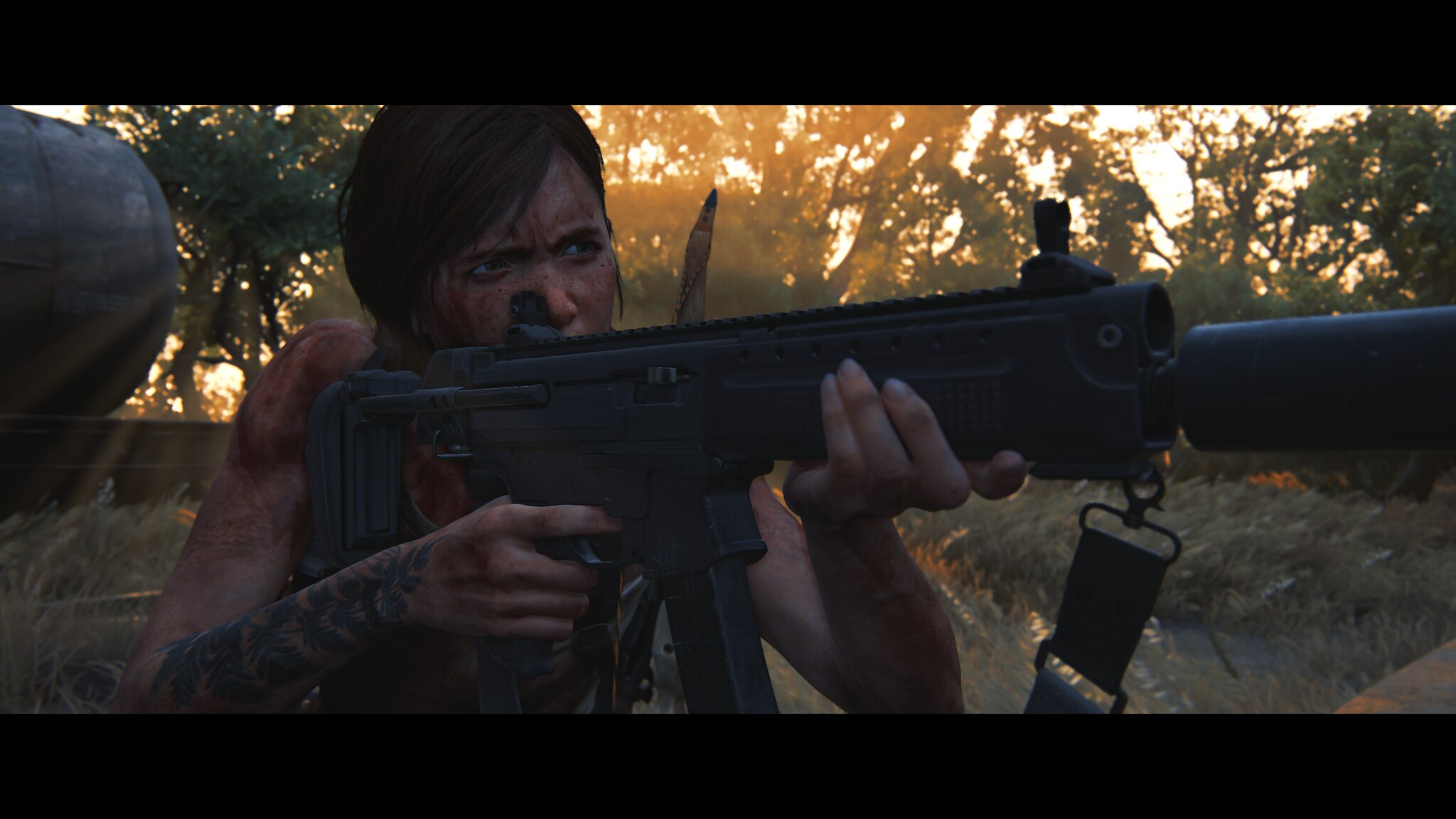In a detailed screenshot from the video game "The Last of Us 2," we see Ellie, the main focus of the image, aiming a submachine gun equipped with a silencer and a strap for shoulder carrying. She holds the gun with both hands, her finger on the trigger, and her intense, squinting eyes indicate she's carefully aiming down the sight, looking quite angry. Ellie appears to be in a wooded area during either dawn or dusk, with the low, golden sunlight streaming through the trees. Behind her, the forest floor is lush with bushes, tall grass, and plants. A metal structure or machine is also visible in the background. Ellie herself is in a disheveled state, her arms bruised, covered in dirt and mud, and adorned with black floral and leaf tattoos. Her somewhat long hair, particularly her long bangs, adds to her fierce appearance. She exudes resilience and determination even in her battered condition.